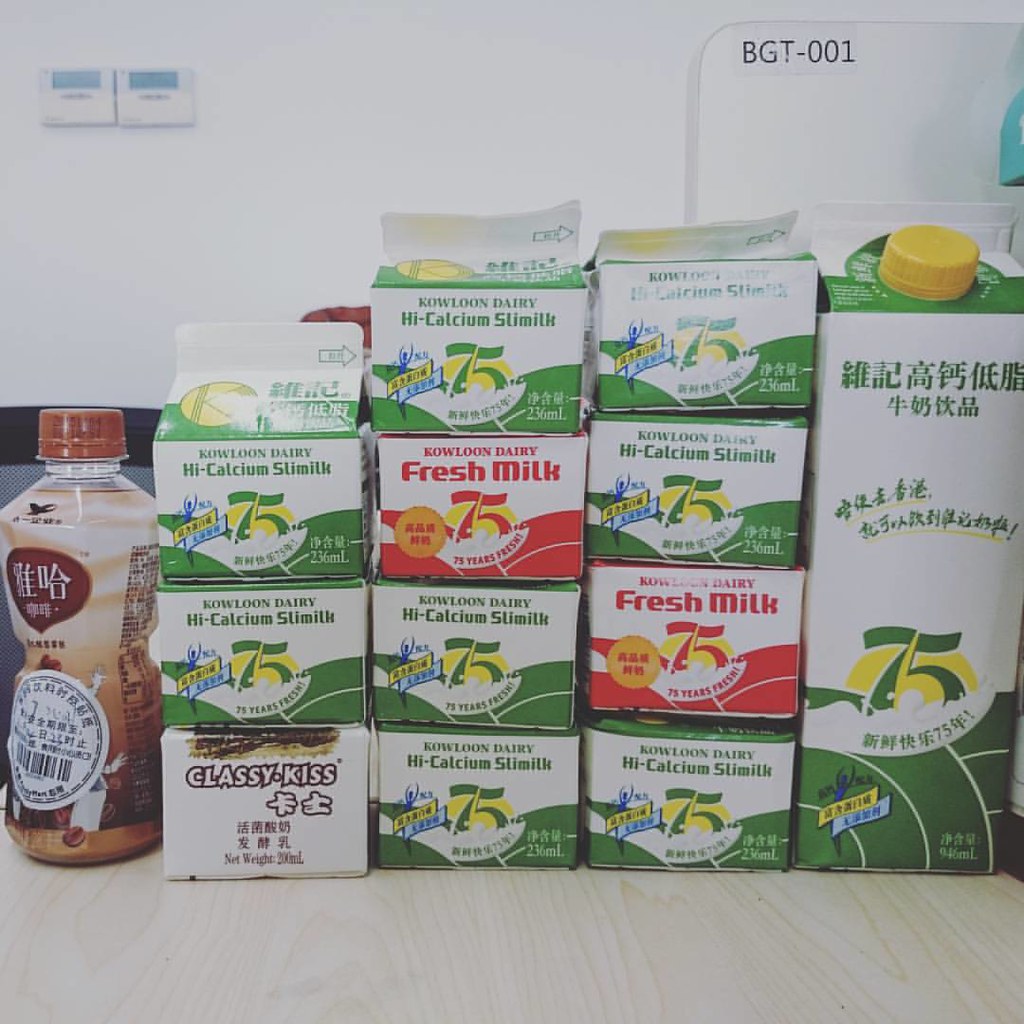The image depicts an organized display of various milk products arranged on a light wooden countertop against a white wall. The arrangement includes four rows of three single-serving milk cartons each, and features distinctively labeled cartons in Japanese. Mixed among them, on the far left is a brown plastic bottle of chocolate milk with a brown cap and white decals. The bottle stands out with its dark brown to creamy colored labeling.

Moving towards the right, the first column contains three half-pint cartons; the bottom one is branded "Classy Kiss" and showcases a white and brown design, while the two above it are green, labeled "Knolloon Dairy High Calcium Slim Milk" with a prominent "75" in the middle.

The second column consists of three cartons: two green "High Calcium Slim Milk" cartons on the top and bottom, and a red "Knolloon Dairy Fresh Milk" carton in the center, displaying "75 years" proudly.

The third column mirrors the second with three green "High Calcium Slim Milk" cartons, interrupted by a red "Fresh Milk" carton in the middle.

The last column features three green cartons and, distinctively, on the very right end, a full-sized milk carton with a red or yellow screw top. This larger carton also promotes “75 years” of the dairy brand. 

In summary, the display combines a variety of small and full-sized cartons, emphasizing the "Knolloon Dairy" brand, with a mix of "High Calcium Slim Milk" and "Fresh Milk" offerings, all detailed in Japanese and English text.